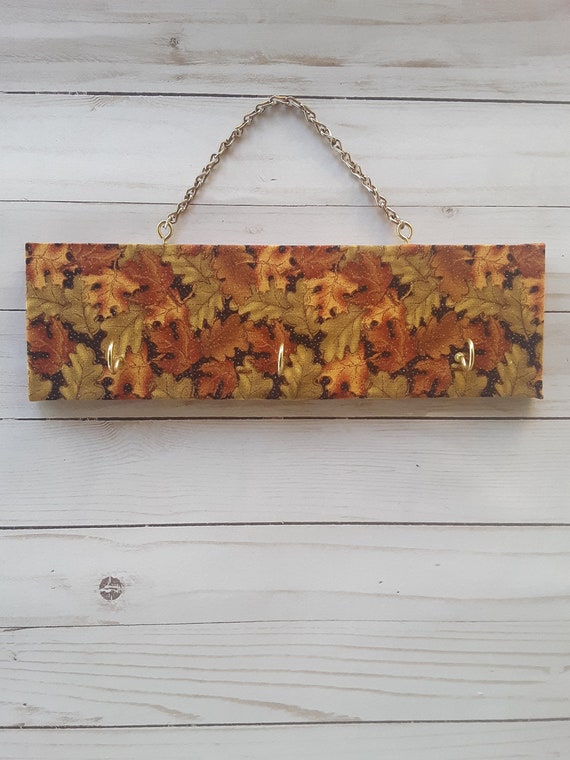This image features a homemade, rectangular coat hanger adorned with a beautiful autumn-themed fabric showcasing vivid fall leaf patterns in shades of orange, green, red, and golden hues. The panel is creatively designed with three chrome hooks for hanging items, subtly integrated into the decorative piece, which adds a touch of functional art to the setting. It is suspended from a whitewashed shiplap wall, reminiscent of barnyard wood, using a bright gold chain that loops through two round links attached to the top of the plaque. The overall scene reflects a cozy, seasonal atmosphere with an emphasis on handcrafted charm and detail.